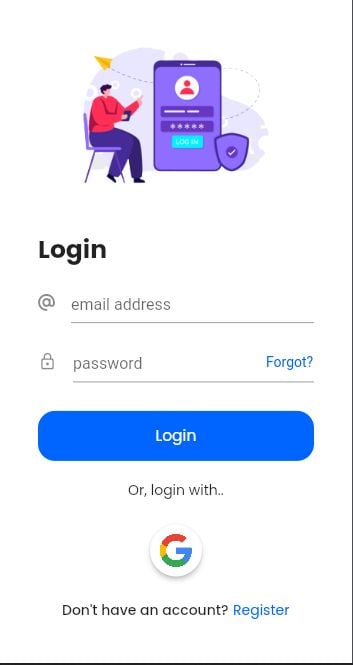This image showcases a login page with a vibrant and modern design. At the center upper portion, a detailed graphic depicts a person wearing purple pants and a red shirt, seated on a purple chair, holding a phone in one hand and pointing with the other. To the right of this figure is an enlarged purple phone with an icon of a person on its screen. 

Below this illustration, there are two dark purple rectangular bars, followed by a teal bar underneath them. Adjacent to these bars on the right is a shield icon. Adding a dynamic touch to the background, a light purple organic shape flows out from the phone on the right side, curling back towards the left, and showcasing a flying paper airplane with a dotted movement trail.

Beneath the graphic, the word "Login" is prominently displayed in large, bold black letters. Following this are fields with an "@" symbol and the text "Email Address," underlined by a horizontal line. Further below, a padlock icon accompanies the word "Password," with "Forgot" placed to the right in blue text. 

Another horizontal line sits beneath, leading to a blue rectangular button with curved corners that reads "Login" in white letters. Alternatively, users can choose to log in via Google, indicated by a circle housing the Google icon and the text "or Login with" preceding it. 

At the bottom, a prompt reads "Don't have an account?" with "Register" highlighted in blue type, inviting new users to sign up.